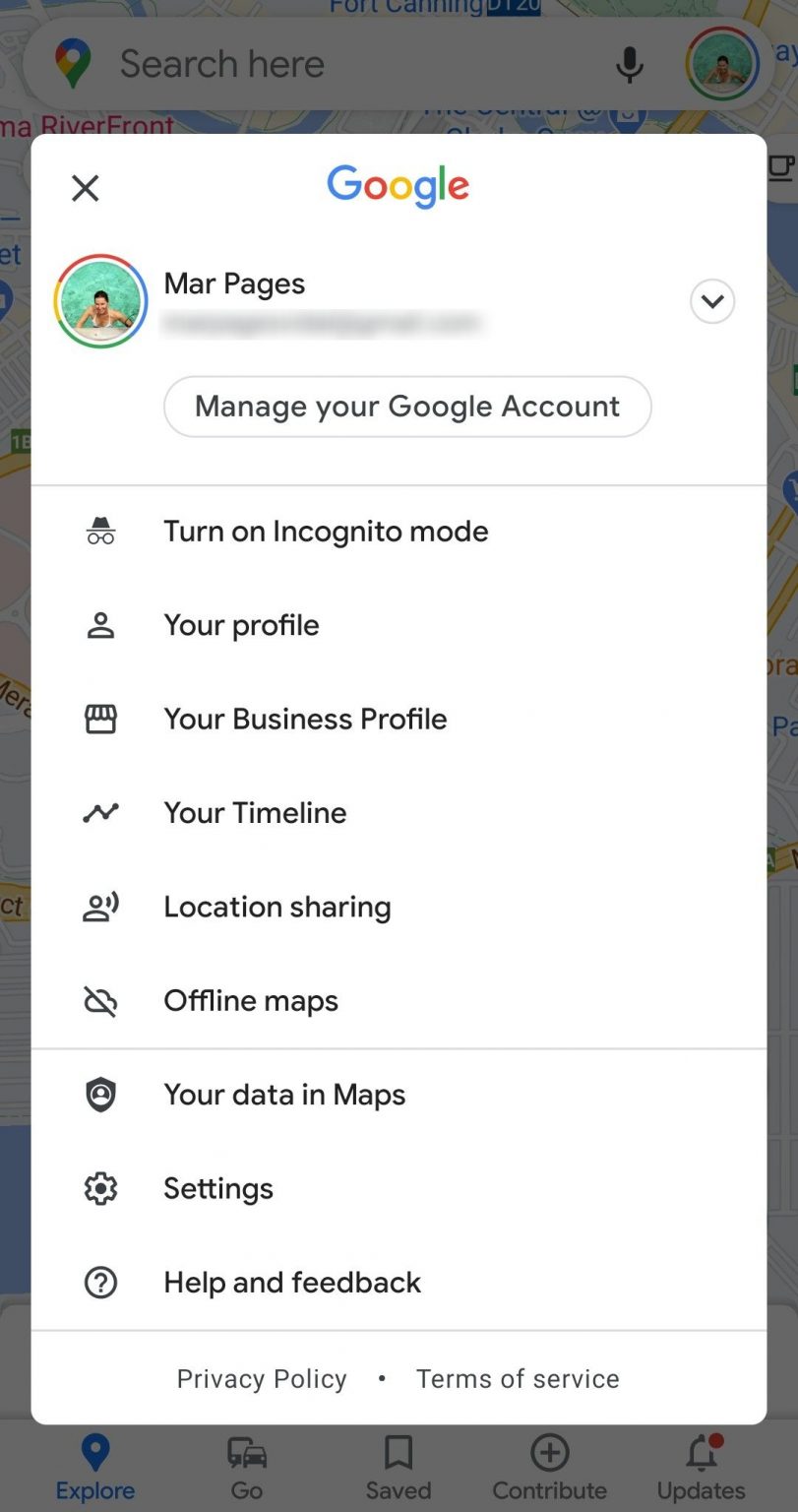This is a detailed screenshot showcasing a user interface of Google Maps with an overlay of the user's Google Account management options. The background features a partially visible Google Maps view with the "Explore" tab engaged, accompanied by prominent colored buttons such as "Go" (paired with a car icon), "Saved" (flag icon), "Contribute" (circle with a plus sign icon), and "Updates" (bell icon with a red dot).

Overlaying this background is a grayed-out section at the top, containing a Google search box distinguished by Google's iconic multicolored pin icon and a gray microphone symbol. To the right, a user profile picture, featuring a person with dark hair in front of a watery backdrop, is displayed.

A pop-up overlay titled "Manage your Google Account" is prominently visible, providing various navigational options: 

- "Turn on Incognito Mode" (complete with a hat and glasses icon)
- "Your Profile" (person icon)
- "Your Business Profile" (storefront icon)
- "Your Timeline" (arrow icon)
- "Location Sharing" (another person icon)
- "Offline Maps" (cloud with a slash through it)
- "Your Data in Maps" (shield icon)
- "Settings" (cogwheel icon)
- "Help and Feedback" (circle with a question mark)

At the bottom of the pop-up are links labeled "Privacy Policy" and "Terms of Service." The screenshot is of high resolution, with clear, bold fonts, and no signs of pixelation or blurring. The email associated with the account is partially obscured for privacy.